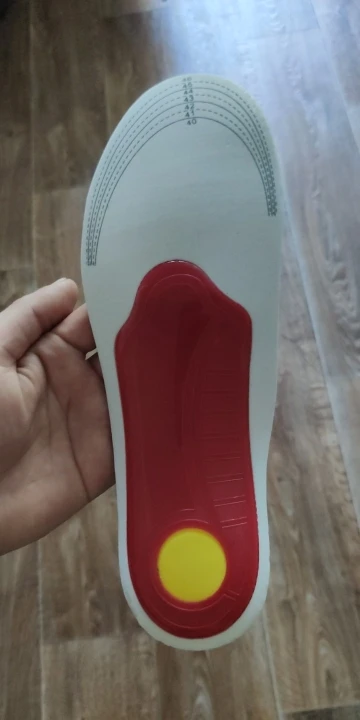In the photograph, an individual is holding a pristine, unused insole for a left shoe in their left hand against a brown-toned wood laminate floor background. The majority of the insole is white, featuring curved, black contour lines at the toe area that serve as a size guide, allowing it to be trimmed to fit shoe sizes ranging from 40 to 46 in increments of 1. The bottom third of the insole, extending from the heel up to about 60% of the insole's length, is equipped with a red rubber or plastic cushioning area. At the very center of the heel, there's a bright yellow circular cushion for additional comfort. The overall scene is sharply focused on the insole, making its detailed design and new, untouched condition the main elements of the image.